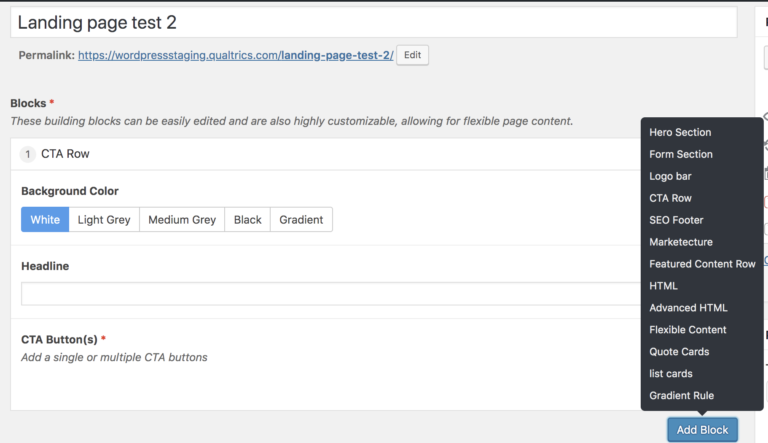The image depicts a testing interface for a landing page, labeled "Landing Page Test 2" in bold black text inside a white rectangular strip. The interface appears on the Qualtrics.com platform, as indicated by the clickable blue-highlighted permalink at the top. An edit button is situated next to the URL for modifications.

The page includes various sections for content customization. Beneath the permalink is a section titled "Blocks," marked with a red asterisk. It features a description in black text stating, "These building blocks can be easily edited and are also highly customizable, allowing for flexible page content."

Further down, a section labeled "CTA Row" specifies that the background color for the Call to Actions (CTAs) is currently set to white, with alternatives like light gray, medium gray, black, and gradient also available. There's a placeholder titled "Place for Headline," where users can input their heading text. Below, another section marked with a red asterisk invites users to "Add a single or multiple CTA buttons."

On the right side, a black sidebar lists various editable components in white text, including:
- Hero Section
- Form Section
- Logo Bar
- CTA Row
- CEO Footer
- Marketer Feature Content Row
- HTML
- Advanced HTML
- Flexible Content
- Quote Cards
- List Cards
- Gradient Rule

At the bottom of this sidebar, an "Add Block" option allows users to insert additional elements into the landing page.